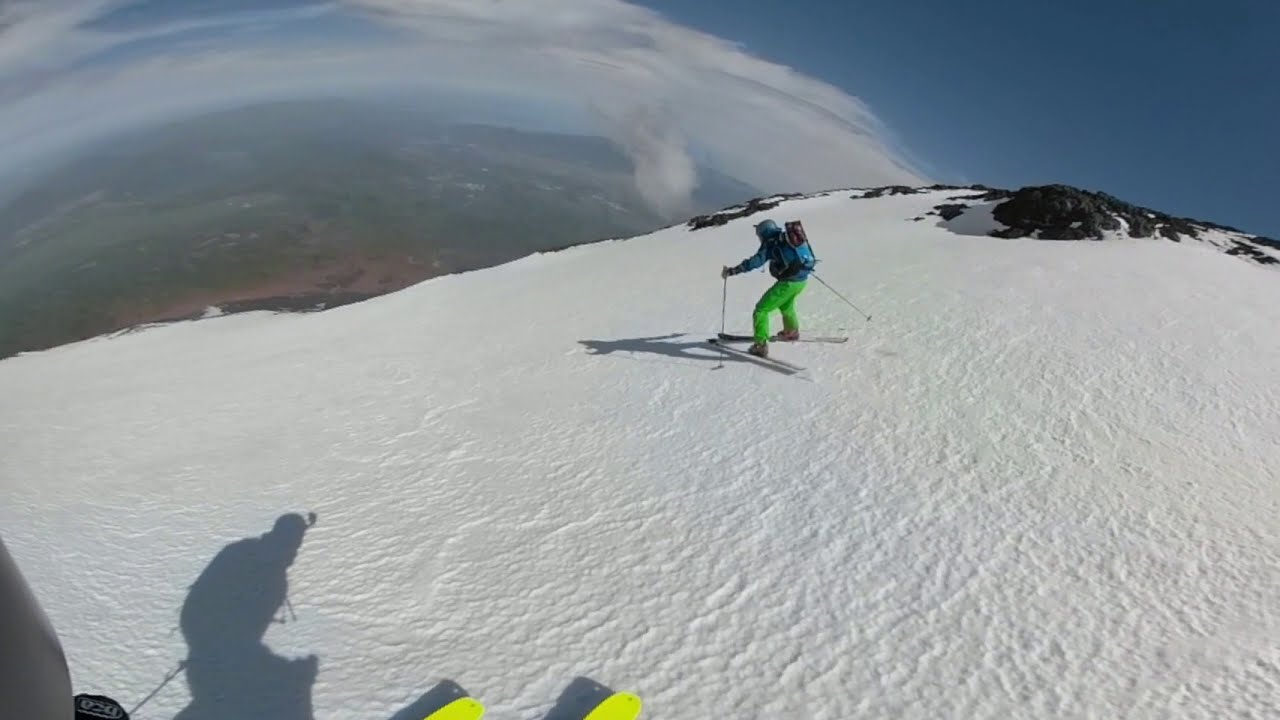The image captures a breathtaking scene of two skiers at what appears to be the summit of an exceptionally high mountain. The central figure is a man in a blue jacket and fluorescent green pants, equipped with skis and ski poles. He's poised on a vast, snowy expanse, almost at cloud level, as indicated by the clouds appearing to arc across the horizon and drift nearby. His green trousers contrast sharply with his dark top and the light blue accents on his backpack. He's also wearing a helmet for safety.

To his right, the mountain's rugged terrain is dotted with black rocks, and above him, the sky is vividly blue. The left side of the image reveals a dramatic drop, presenting a bird’s eye view of indistinct green and brown land far below—an indication of the altitude. The curvature of the horizon emphasizes the incredible height from which the photograph was taken.

On the lower left, the shadow of another skier is visible, along with the fluorescent yellow tips of their skis. This shadow belongs to the person taking the picture, who stands slightly behind and closer to the presumed cliff. Despite the possibility of this being a ski slope, the sheer drop and positioning suggest a cliff edge, adding a sense of danger to the scene. The entire composition underscores the awe-inspiring yet perilous beauty of high-altitude skiing.